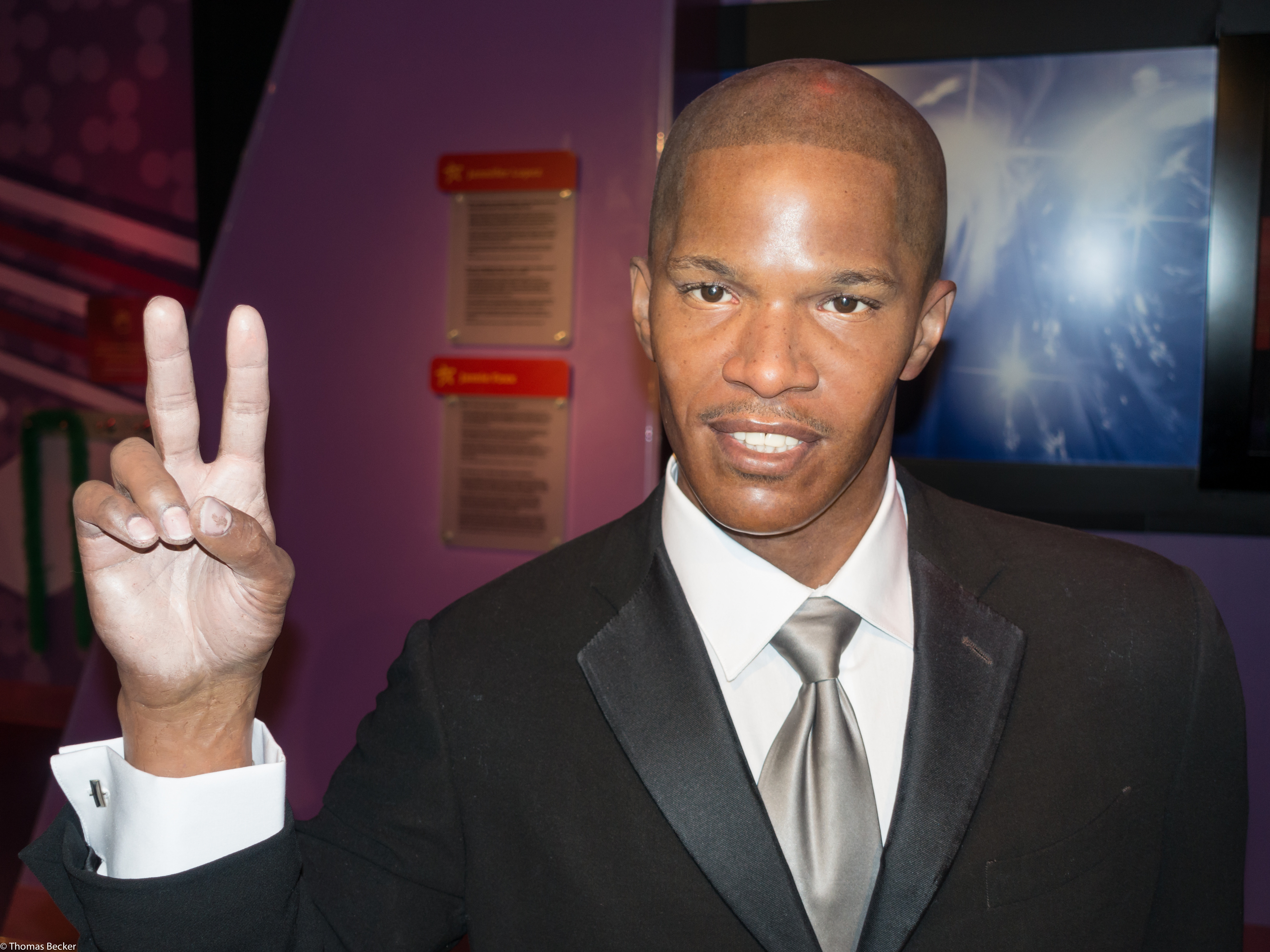The image portrays a figure resembling the actor Jamie Foxx, likely a wax museum subject or an AI-generated figure due to its uncanny valley effect. The scene is framed indoors, showing Jamie Foxx from the mid-chest up, against a purple wall. He has medium-brown skin and a very closely shaven head, revealing a faint hairline. His expression is neutral with slightly parted lips, displaying both rows of teeth and a subtle mustache. Foxx's gaze is directed downwards and to the left. He dons a black suit jacket with a silk lapel, a crisp white dress shirt, and a silver tie. His right hand is raised in a peace sign, with his thumb touching his ring and pinky fingers, and his index and middle fingers extended. Notably, his palm and fingers appear to have chalk on them. The background features a blue screen embedded in the purple wall and two plaques with red headers and gold stars, though the text is indiscernible. Additionally, there is some shelving visible towards the left, enhancing the scene's indoor setting. The lower-left corner of the image includes the copyright mark "© Thomas Becker."